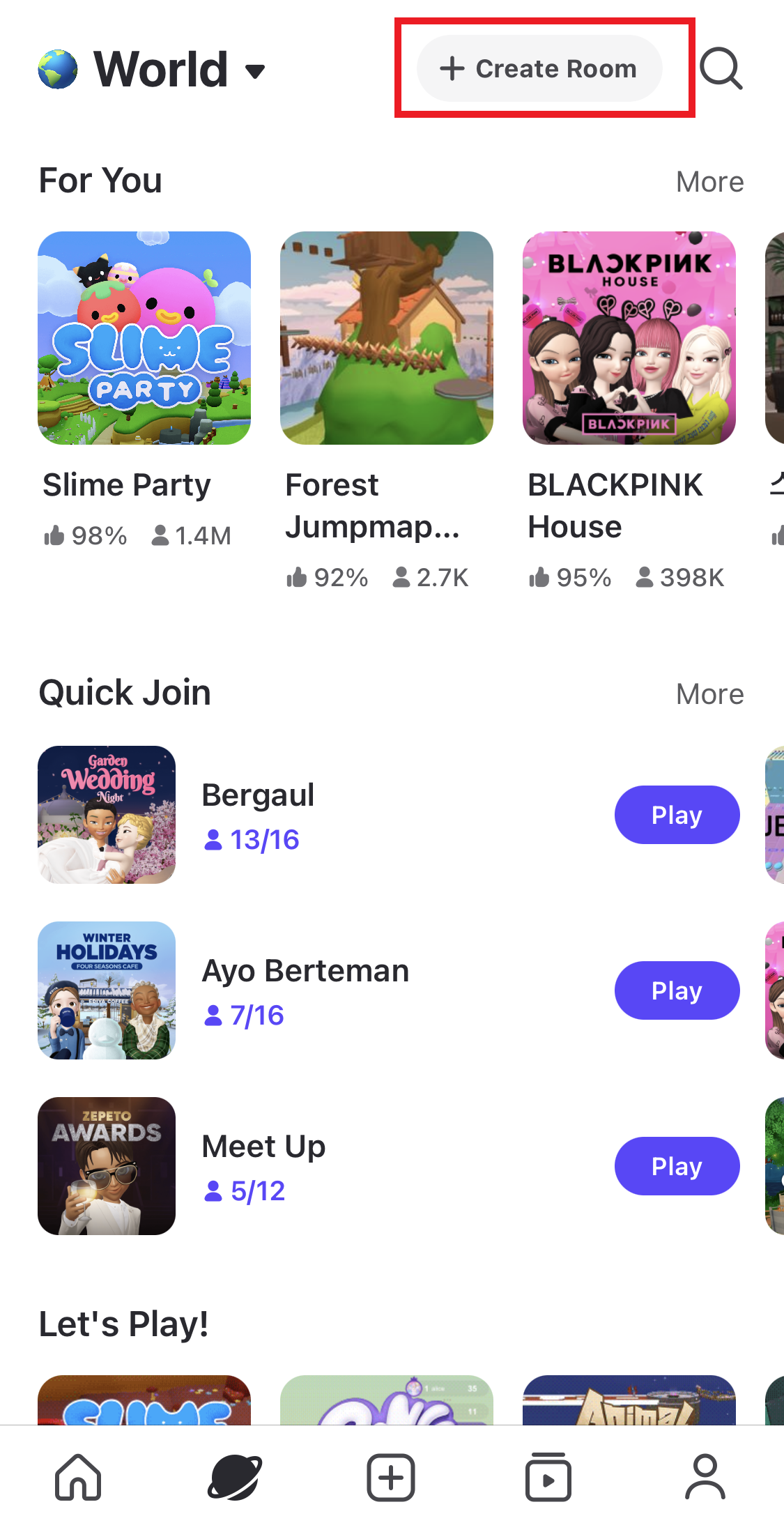The image appears to be a screenshot of a smartphone interface. In the top-left corner, there is a globe icon labeled "World" next to a red-outlined rectangle that says "Create Room." Beside these elements is a search icon. Directly below this section, there's a label "For You" followed by a set of three squares, each displaying different anime-themed images.

1. **Slime Party**: The first square features a game called "Slime Party," depicting a relevant image.
2. **Forest Jump Mat**: The second square showcases an image of a small house on a grassy hill, labeled "Forest Jump Mat."
3. **Black Pink House**: The third square includes an image of four anime girls with the label "Black Pink House."

Underneath these squares, there's a "Quick Join" section displaying three emblems labeled "Wedding," "Holidays," and "Awards," each accompanied by a blue play button.

Towards the bottom-left of the interface, the text "Let's Play" is visible, leading to another section with three more games. The top game, labeled in light blue, is called "Slime." The second game is in gray but its name isn't visible. The third game, in dark blue, is partially visible and labeled "Animal."

The layout appears user-friendly, offering quick access to various themed games and activities.